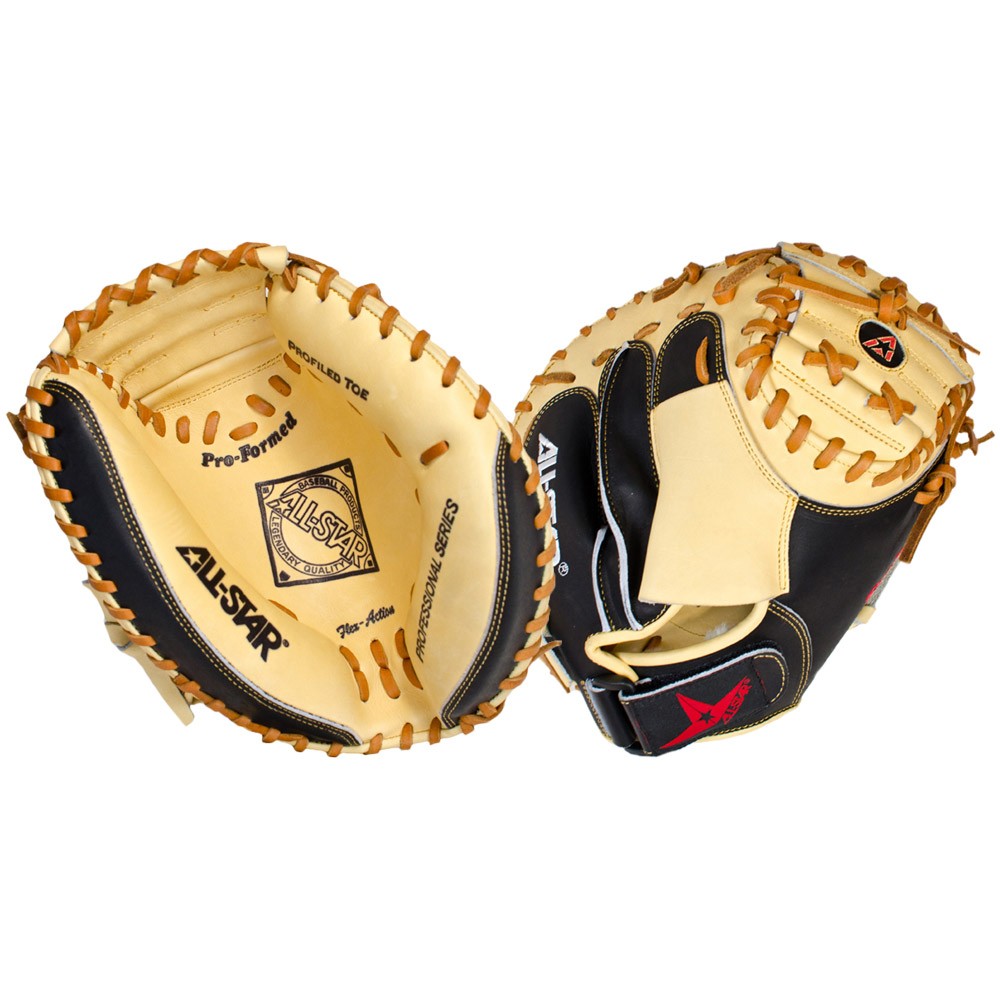The image displays a detailed, close-up view of a catcher's mitt against a completely white background. The mitts are positioned side by side, showcasing both the front and back. The left side of the image features the front of the catcher's mitt, predominantly in a light tan color with dark brown stitching and a black edge. In the center of the mitt, within a black diamond, the word "All-Star" is prominently displayed. Additional black text on the front includes "Professional Series" on the right side and "Proformed" at the top.

The right side of the image reveals the back of the mitt, which has finger slots made of black leather and a continuation of the light tan coloring. The mitt's webbing includes a small circular black area with a black star in the logo. There is also a black Velcro adjuster labeled "All-Star" in red. The intricate design and varying colors of the mitt's materials, including the black leather trim and light brown stitching, highlight the sophisticated craftsmanship of this professional catcher's mitt.